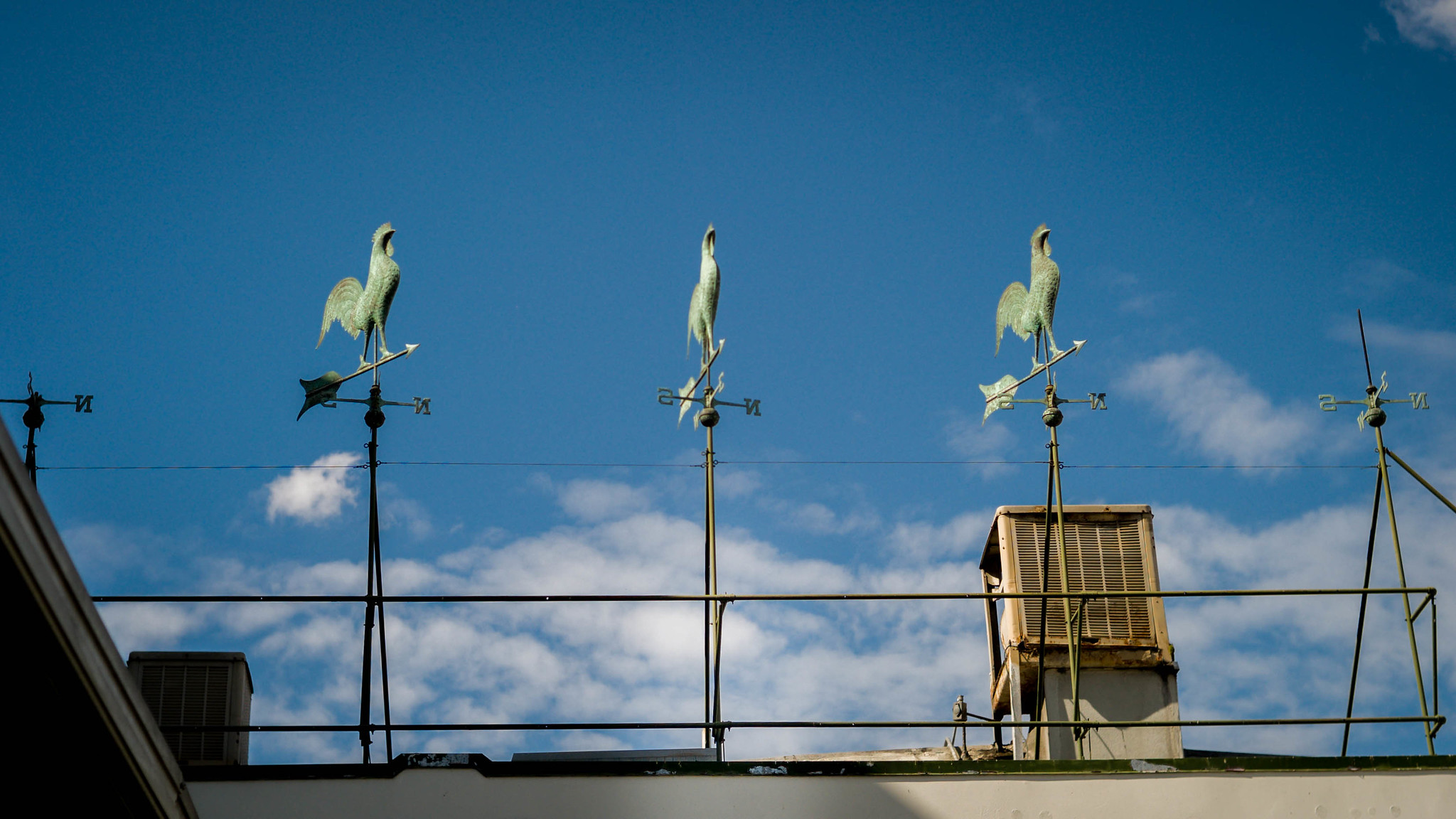The photograph captures the edge of a flat rooftop adorned with a series of five weather vanes under a bright blue sky dashed with pillowy white clouds. In the center, three prominent weather vanes each bear a green, slightly discolored rooster. The two roosters on either side are aligned, pointing to the right, while the central rooster faces almost head-on toward the viewer. Flanking these roostered weather vanes are two simpler weather vanes, each missing the rooster figure but marked with directional indicators for north, south, east, and west. Behind one of the rooster-topped vanes, a rusty beige mechanical unit resembling an air conditioning or heating unit with a ventilated grill stands out. Nearby, additional light gray AC units rest on concrete and steel posts. Surrounding the scene is a simple steel railing, constructed from welded pipes, encircling the rooftop.